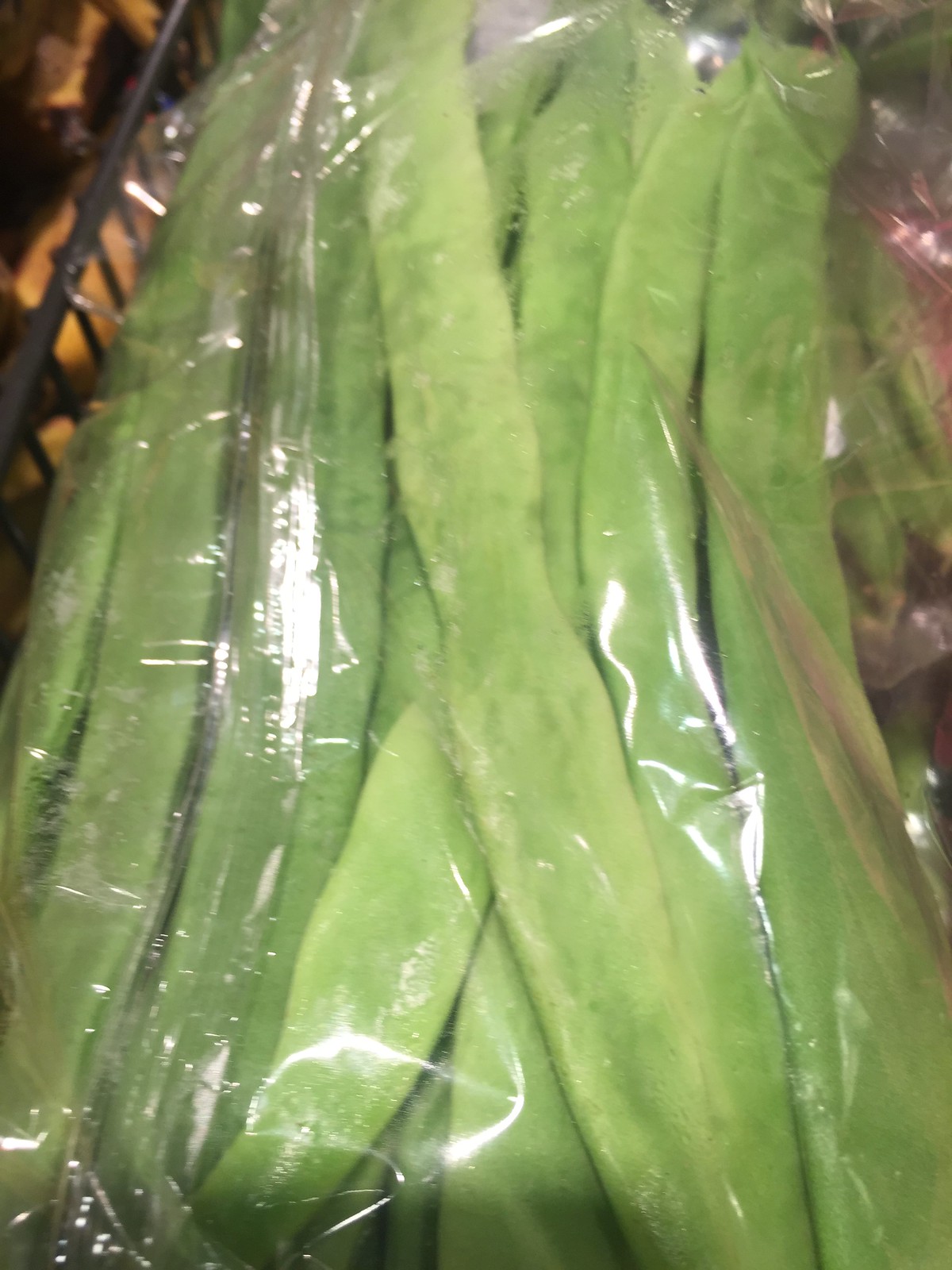This photograph captures a close-up shot of a large bag of long, pale green string beans, still in their pods, enveloped in clear plastic wrap. The bag has a sheen, likely from the camera flash, suggesting it's tightly wrapped. The scene appears to be set inside a black shopping cart, hinting that someone is shopping for produce. The yellow bowl initially mentioned is less discernible, but the dominant setting remains the shopping cart. Off to the upper left-hand corner, other food items can be faintly seen between the cart's bars. Despite their plain appearance, the fresh string beans look enticing, as if ready to be purchased and cooked for a meal.